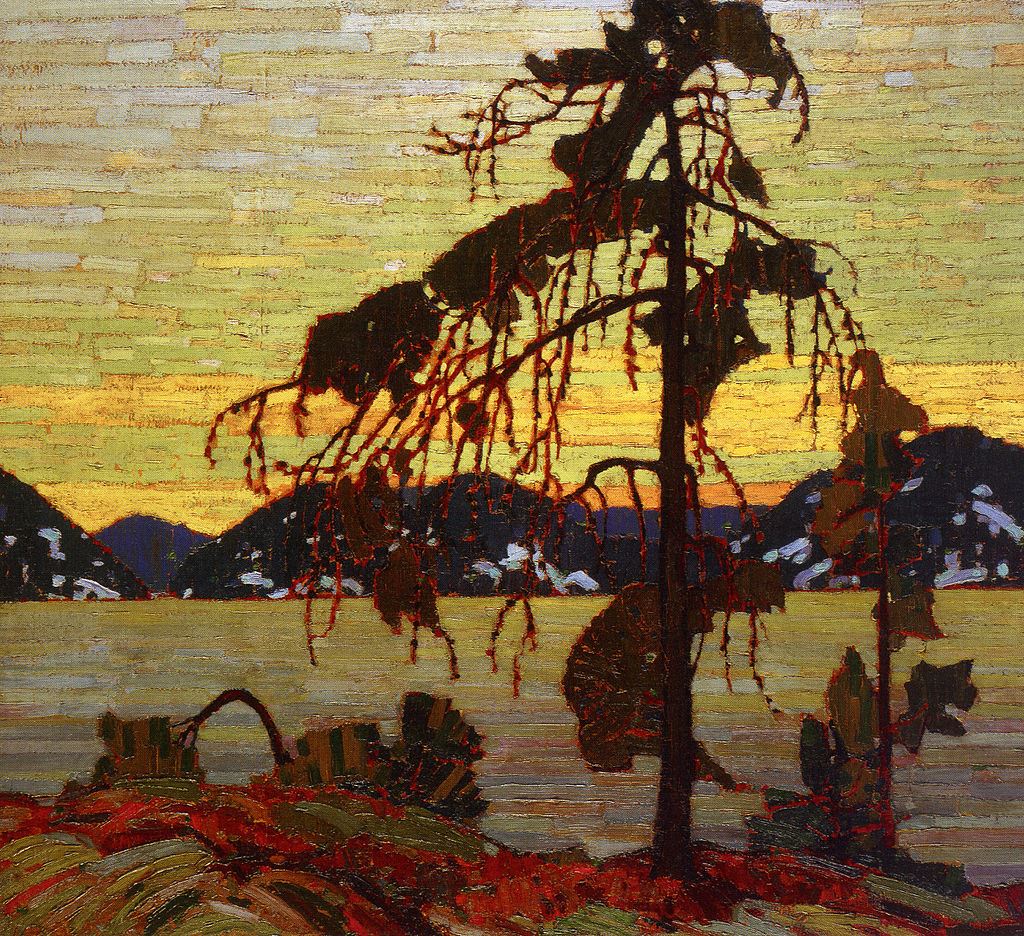This artwork, seemingly a photograph or scan of a painting, depicts a melancholic yet vibrant scene showcasing a dying tree situated on the right side of a riverbank or lakeshore. The central focus is a partially barren tree with a long brown trunk whose drooping, red-tinged branches suggest a bleeding effect, enhancing its desolate appearance. The few remaining leaves are brown and misshapen, emphasizing the tree's diseased state. Nearby, a broken branch lies discarded, and a much smaller, similar tree struggles to grow beside it. The backdrop features a large body of water extending towards distant, dark mountains. Beyond these are even further mountain ranges, capped with snow, juxtaposed against a poignant sky transitioning from deep orange near the horizon, through yellow, to a pale hue as it rises. Despite the rich colors, the overall darkness and the unhealthy state of the tree impart a somber, almost hopeless, mood to the artwork.